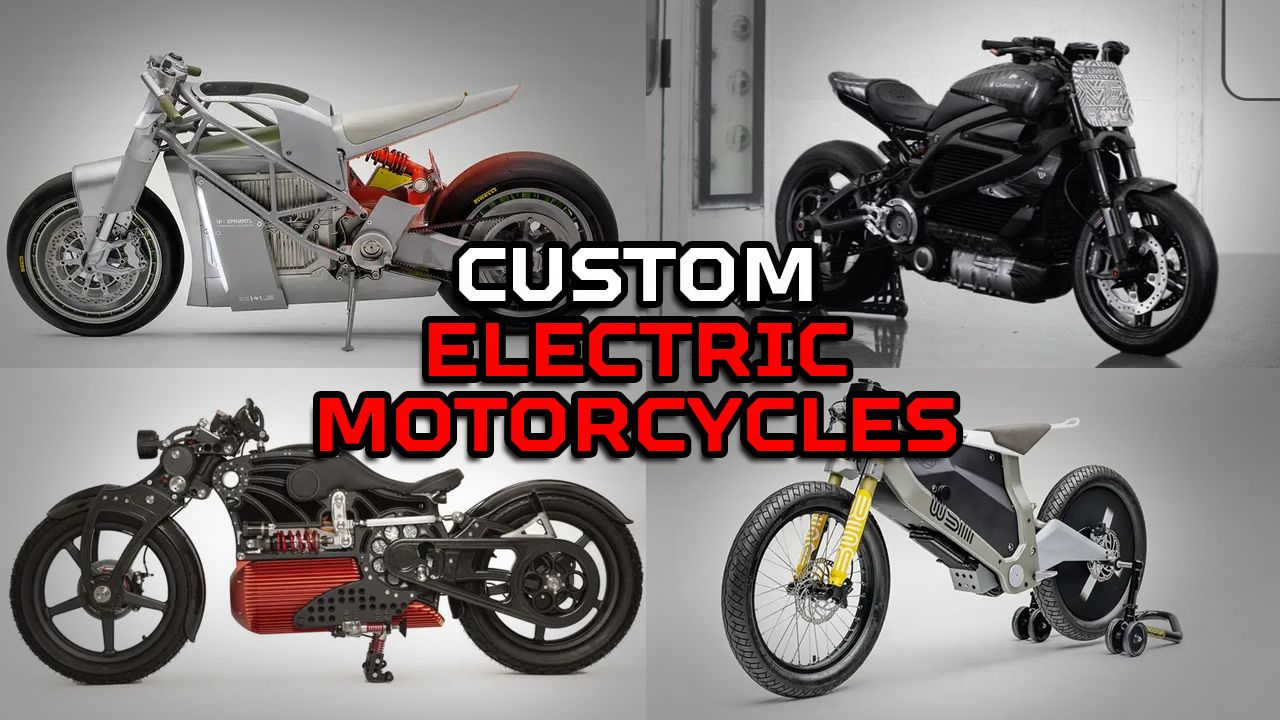The image features four distinct pictures of custom electric motorcycles arranged in a 2x2 grid, each with even spacing. At the center, in white and red bold capital letters with a black outline, the text reads "CUSTOM ELECTRIC MOTORCYCLES." 

- The top left quadrant showcases a mostly white motorcycle with a red engine below the seat and some yellow detailing near the rear wheel. This bike is oriented to the left.
- The top right quadrant displays an all-black motorcycle with a large headlight and silver trim, facing to the right.
- The bottom left quadrant features another black motorcycle with a red barrel-shaped component near the spokes and pedals, also oriented to the left.
- The bottom right quadrant portrays a futuristic-looking gray motorcycle with thin wheels and some yellow bar detailing. This motorcycle appears to have additional stability support, resembling training wheels. 

Each motorcycle is unique in design, highlighting the variety and customization possible in electric motorcycles.